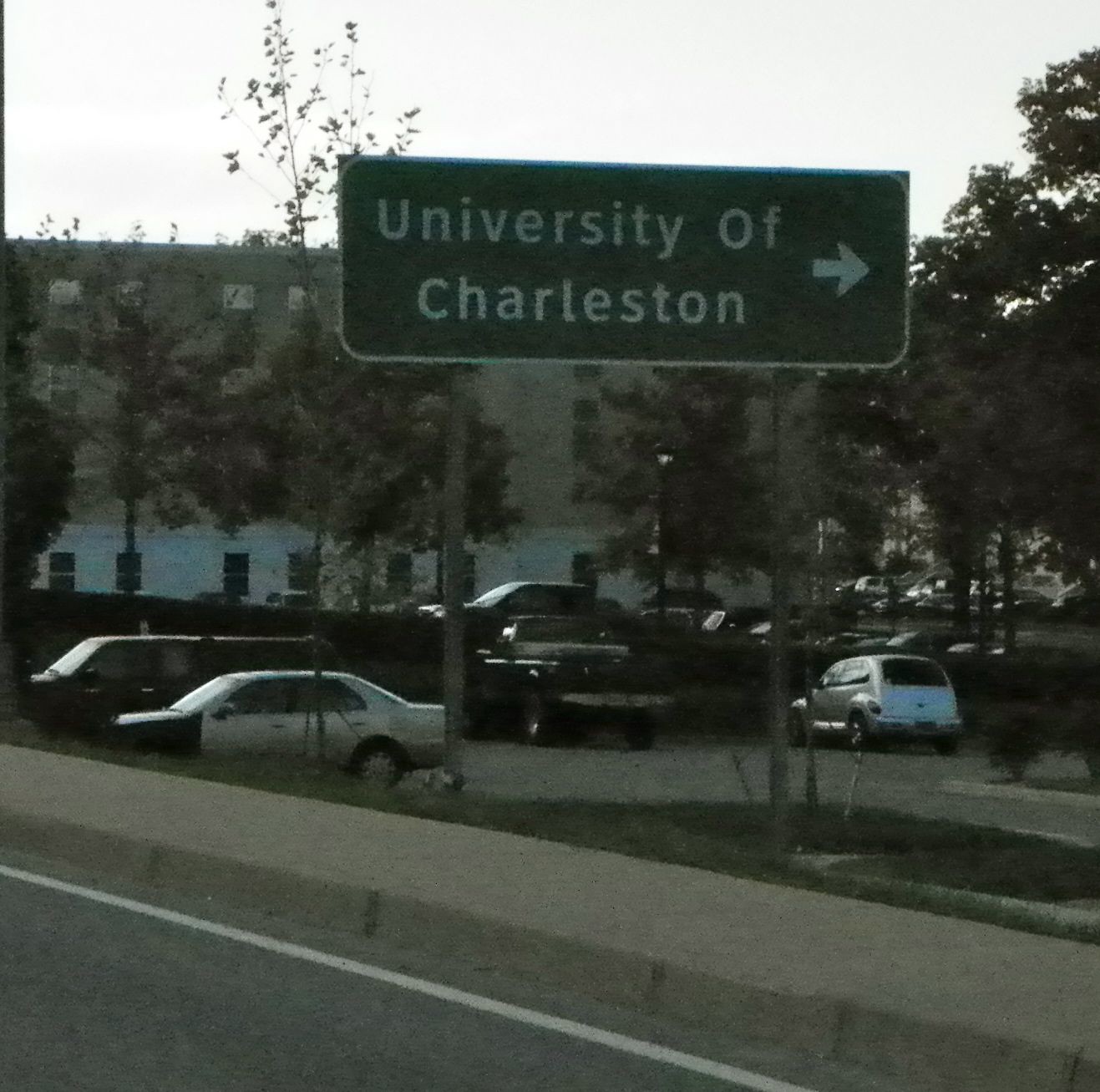In this photograph, the focal point is a prominent sign displaying "University of Charleston" with an arrow directing to the right. The scene captures a bustling parking lot featuring various vehicles, including a truck, several sedans, and a notable pickup truck with a cap on its back. In the background, an imposing building, likely part of the university campus, stands tall amidst the landscape. Trees adorn the parking lot and the perimeter of the building, adding natural charm to the setting. The foreground showcases a street marked with a white line that typically delineates the shoulder, although in this instance, it transitions into a sidewalk. Verdant grass frames the lower part of the image. The predominant hues in the photograph are shades of green, tan, and the striking contrasts of black and white.